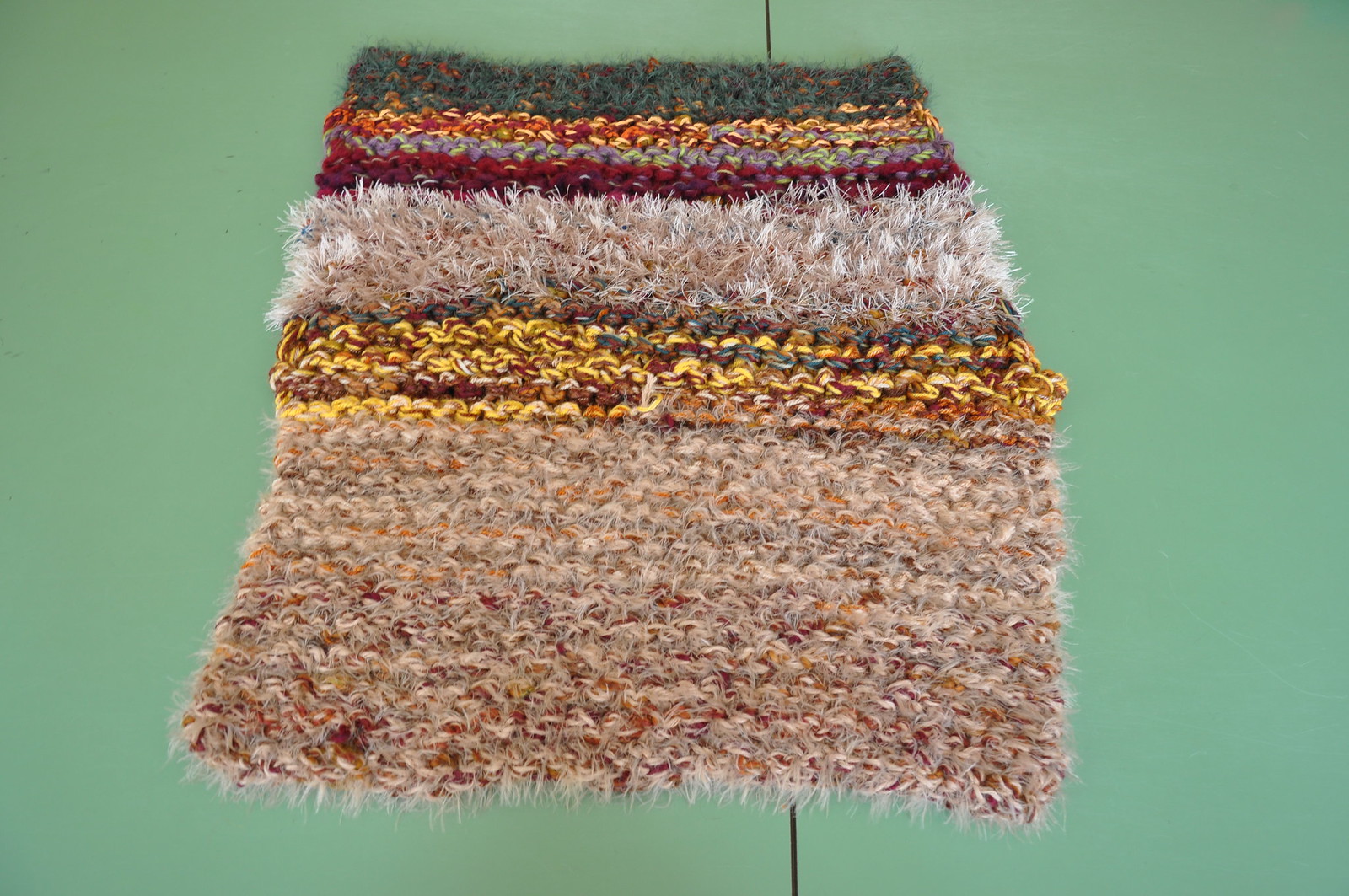This image displays a close-up view of a colorful knitted fabric set against a teal green background. The fabric, which could be part of a handmade dog sweater or another knitted garment, appears fuzzy and textured, characteristic of wool or yarn. The piece has a roughly square shape, although it is not perfectly even, with small openings at the top and a larger one at the bottom.

From top to bottom, the knitted fabric features several distinct horizontal stripes. The topmost stripe, approximately an inch wide, is green with small hints of red. Below it is another inch-wide stripe of yellow mixed with some red. The next stripe is a thin band of purple and green. Following that, there is a red stripe that includes a few pinkish areas and some black dots. This is succeeded by a notably fuzzy section that appears white and brown, tapering from white at the tips to brown towards the base.

Further down, a broader stripe combines red, blue, and orange in a slightly chaotic mix. Below this, a fuzzy stripe composed of dark and light browns occupies about an inch; it resembles the texture of house carpet. The final section of the fabric blends blue-gray, brown, and red tones, interspersed with tan and yellow. Running vertically through the fabric is a gray thread or string, adding another layer of texture and detail to the piece. Overall, the image showcases an intricately knitted, colorful item with varied textures and hues.